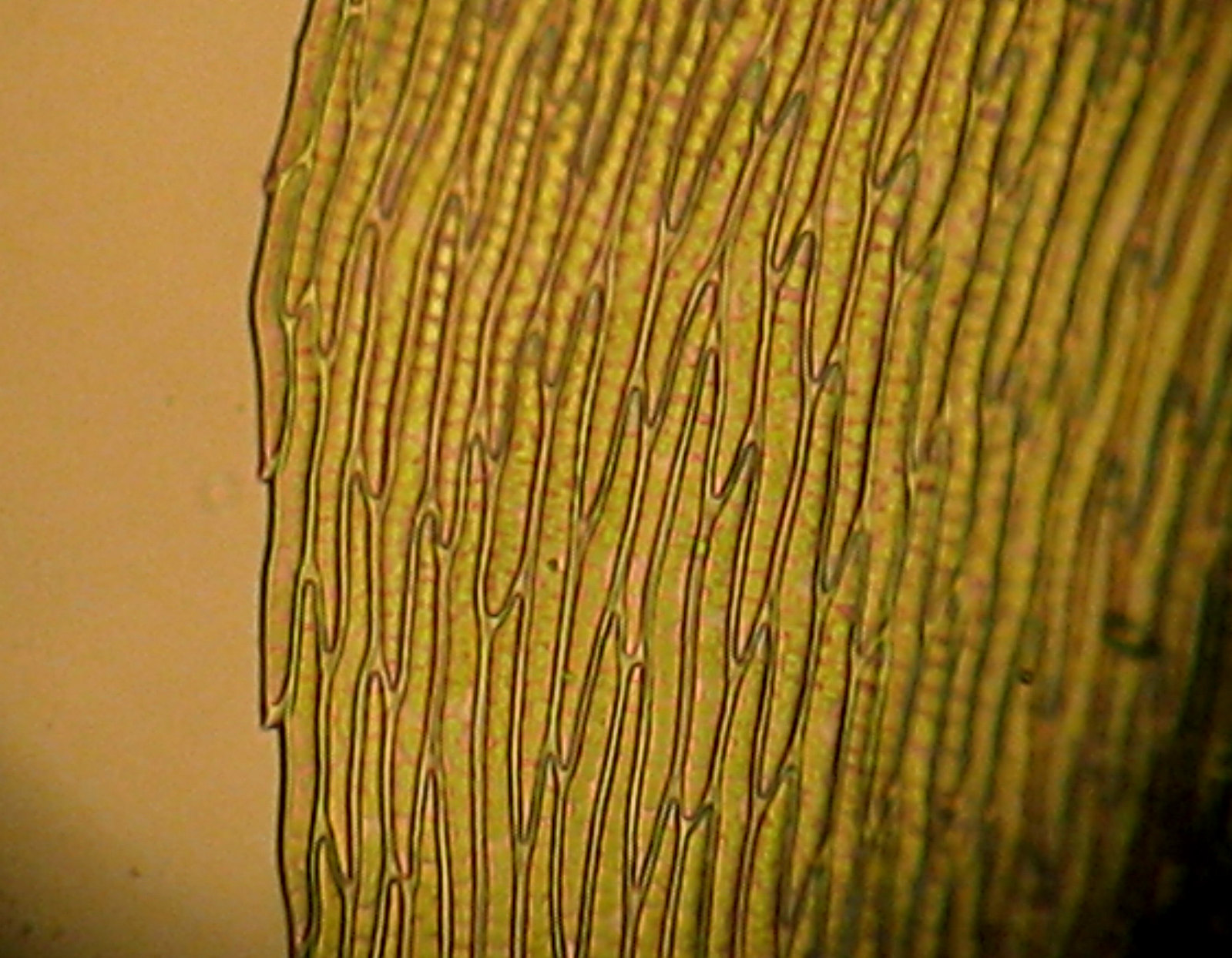This image captured under a microscope reveals an extreme close-up of plant cells, showcasing their characteristic green hue and elongated, flat structure. The cells are densely packed together, each one distinctly defined by its cell wall. Light interactions create a psychedelic effect with rainbow distortions as it passes through the translucent cell material. A notable feature within the cells is the visible chlorophyll, interspersed with slightly pink areas. The background fades to a tan color, with vertical, yellowish strips adorned with dark and pink striations filling the right side of the image. The overall composition suggests an artistic quality, but the overwhelming presence of plant cells grounds it in a biological context.